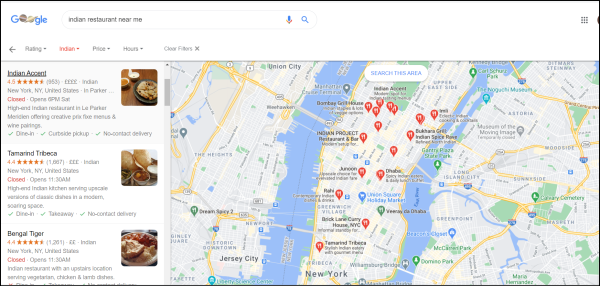Sure, here's a cleaned-up and detailed descriptive caption for the given image:

---

The image is a screenshot of a Google Maps search result for "Indian restaurant near me." The interface includes the recognizable Google logo in the top left corner, featuring the multi-colored letters in blue, red, yellow, and green. Adjacent to the logo is a light gray search bar with dark text displaying the search query. To the right of the search bar, there is a blue microphone icon with a red base, a magnifying glass for initiating the search, and an icon resembling a square with nine black dots arranged in a grid, presumably for accessing additional apps or features.

Below this upper interface, there's a row of options on the left side, including a gray arrow pointing to the left for navigation, the word "Rating" with a period after it, and red text with downward arrows for "Print," "Hours," and "Clear Filters" followed by an 'X' icon.

The results section displays details for three Indian restaurants. Each listing includes the restaurant's name, star rating in orange, and pertinent information such as hours (with the word "Closed" in red if applicable), phone number, and icons indicating the availability of dine-in, customer pickup, and delivery services (though the delivery text is not entirely legible).

1. The first restaurant has four and a half orange stars, and its details include its operating hours, contact information, and a note that it is closed at the moment. Green checkmarks indicate available services.
   
2. The second restaurant, "Tremead Tarabecca," has a 4.4-star rating and similar details, including a red "Closed" indicator.

3. The third restaurant, "Bengal Tiger," also has a 4.4-star rating with the same format of information.

Each listing is accompanied by a small square image of the restaurant or its food offerings.

The majority of the right-hand side of the image is occupied by a map view, highlighting the locations of various restaurants with teardrop-shaped markers. Most markers are red, indicating the type of locations searched for, with a few blue and green markers sporadically placed.

---

This caption provides a comprehensive description of the screenshot, detailing the interface, search results, and map features.